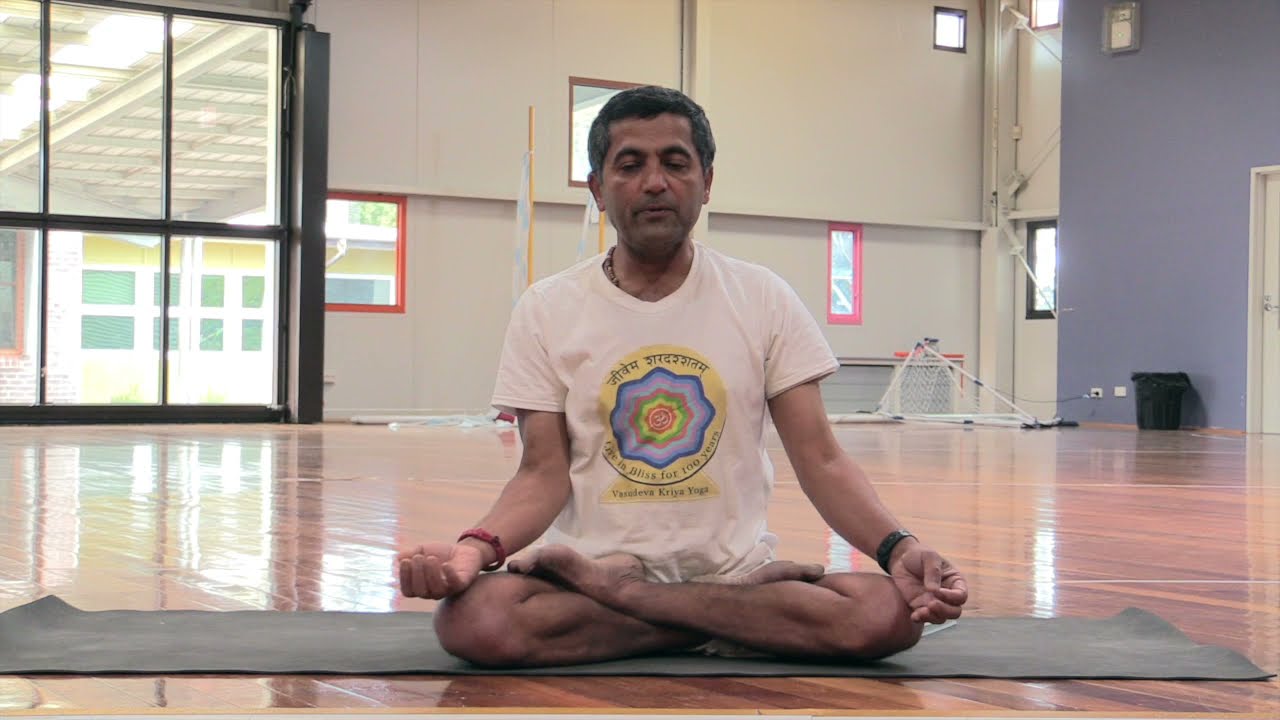A medium-skinned man, aged around 40 to 50, is meditating in a serene gym environment. The gym features a shiny wooden floor and a long gray yoga mat on which the man sits in a yoga pose with his legs crossed and his palms facing up, eyes closed in deep focus. He is dressed in a white t-shirt adorned with a vibrant design featuring a yellow circle with a multi-colored blue, orange, green, yellow, and red flower in the center, and text in black, which hints at an Indonesian alphabet, reading "Give in bliss for a hundred years." The man also wears a watch on each wrist and a red bracelet. Behind him, the gym’s white wall is punctuated with several large windows, allowing sunlight to flood the room. The gym's architecture includes a wall on the right side painted in a light purple or lavender hue, and to the left, a series of windows with blue and black steel frames.